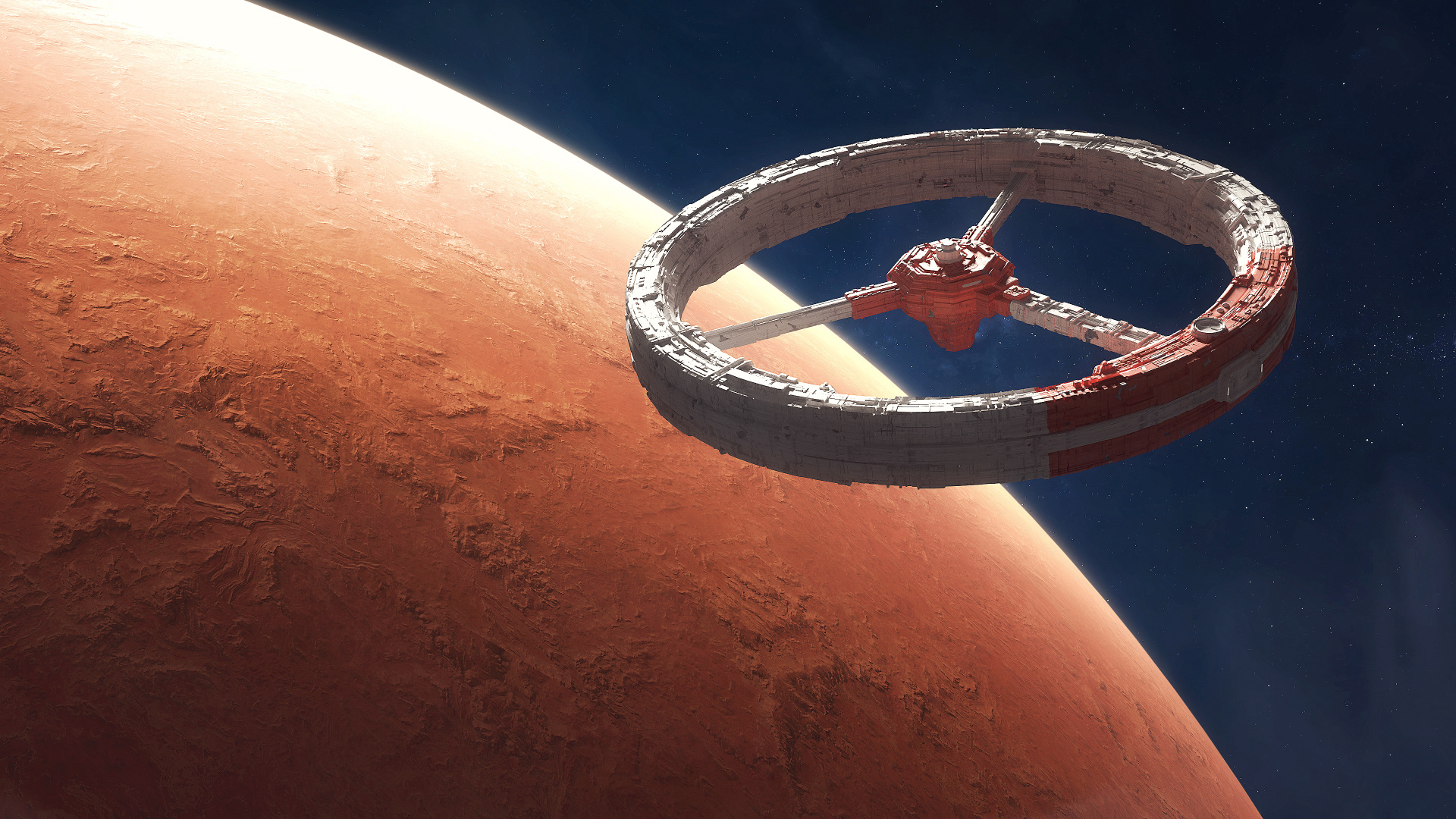The image depicts an artistic rendering of a space station orbiting Mars, evoking a scene reminiscent of Star Wars. The central feature is a spacecraft shaped like a horizontal wheel, segmented into thirds by three support beams, akin to a pie chart. It has a distinct red center with red stripes along its sides and an overall white and orange hue. The spacecraft’s intricate design and sizeable scale are evident from its detailed textures. Mars, the dominant feature in the background, emerges from the lower left corner, showcasing its characteristic rusty orange surface, complete with visible ridges and mountainous terrain. The planet is bathed in sunlight, illuminating it from the top left to the bottom right, creating stark contrasts and emphasizing its rugged landscape. Surrounding the scene is the vast expanse of outer space, painted in deep navy blue and black hues, interspersed with hazy white areas and twinkling stars, adding to the sense of vastness and isolation.